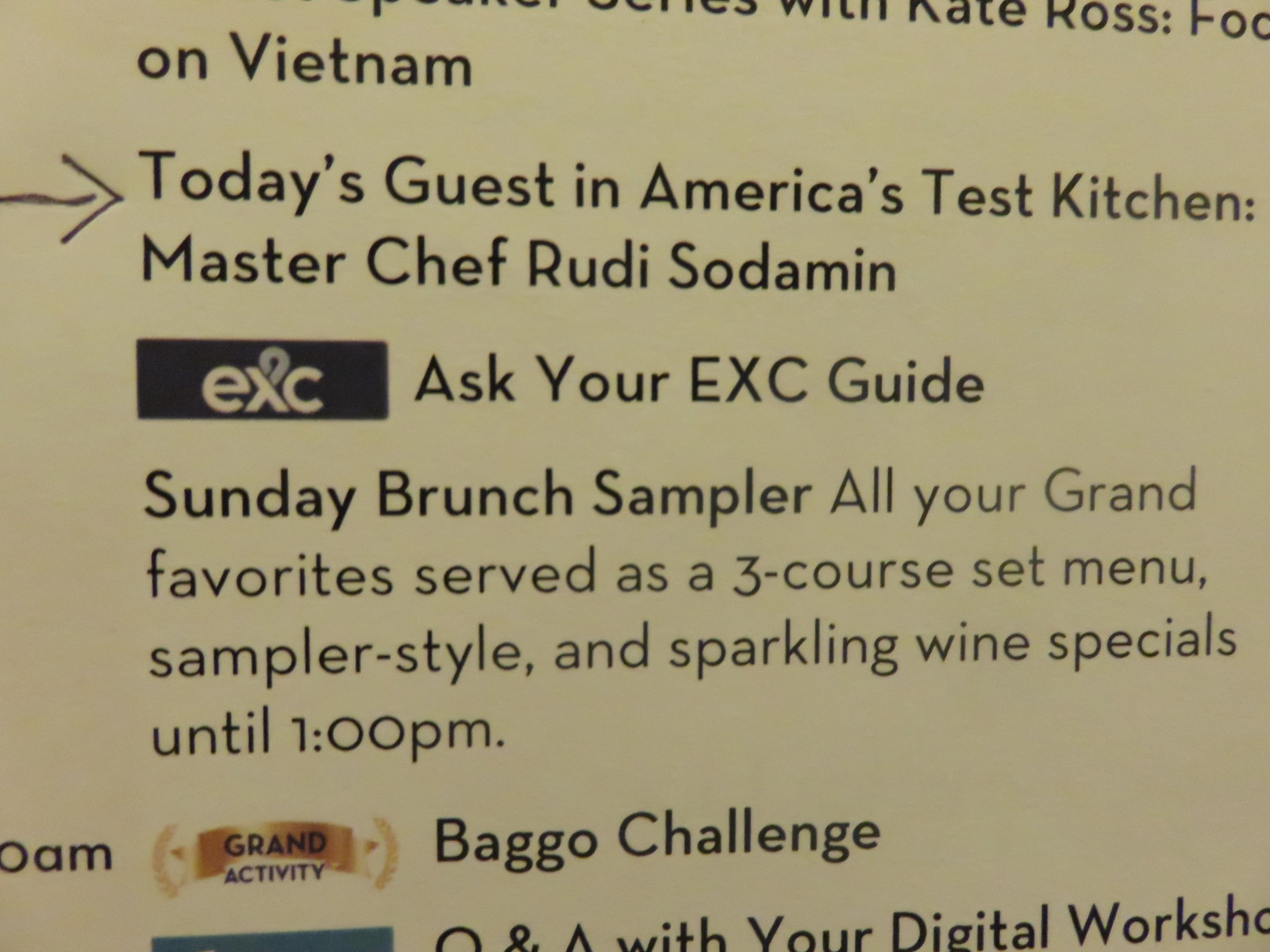The image is a color photograph in landscape orientation, showcasing a close-up view of a program guide for a cooking or menu challenge. It features black text against an olive background, with some portions at the top and bottom cut off. The prominent section has a handwritten arrow pointing to the text "Today's Guest in America's Test Kitchen: MasterChef Rudy Soderman." Below this, there is a rectangular black logo with the white letters "EXC," accompanied by the text, "Ask Your EXC Guide." Further down, a paragraph describes a "Sunday Brunch Sampler" offering "all your grand favorites served as a three-course set menu, sampler style," along with sparkling wine specials available until 1 p.m. Below this description, a gold banner logo stating "Grand Activity" is visible, followed by the text "Bagel Challenge," with more details cut off. The hazy text partially visible above the featured information reads "On Vietnam." This detailed setting suggests a well-planned, enjoyable afternoon filled with culinary activities.